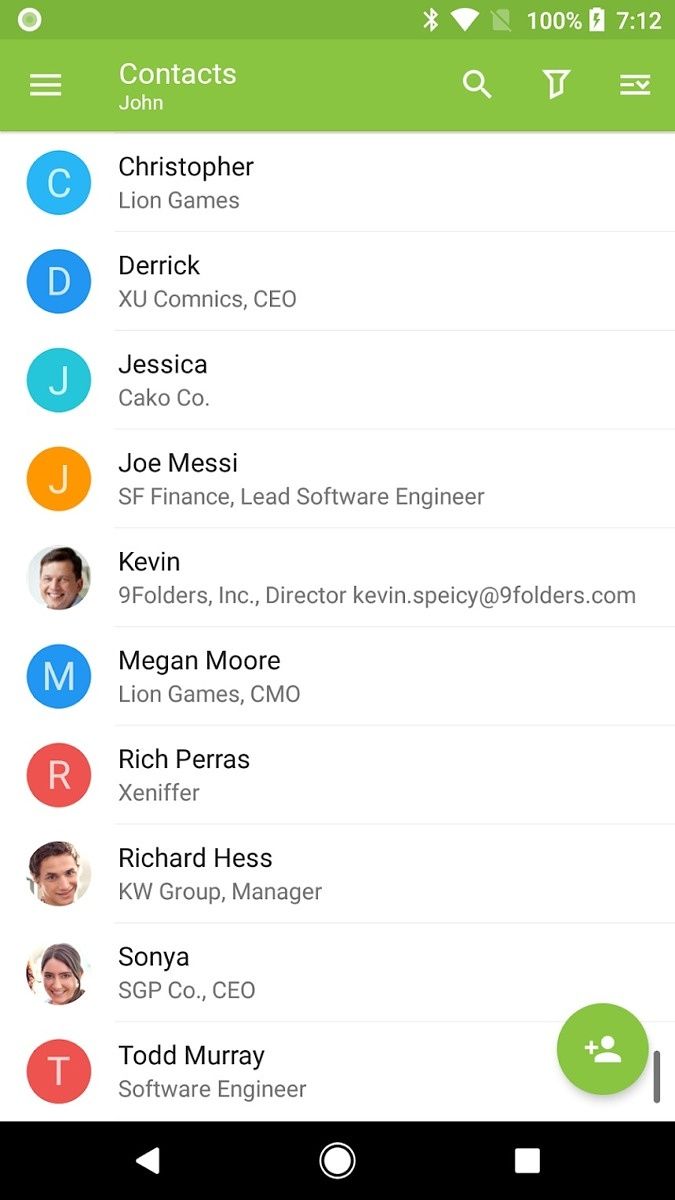The image displays a screenshot of the contact page from an Android device. It shows detailed information including a profile picture, the contact's name, phone number, email address, and various interaction options like call, text, and email. The layout is characterized by a clean, user-friendly interface typical of many Android devices, with distinct icons and options arranged methodically for easy access.